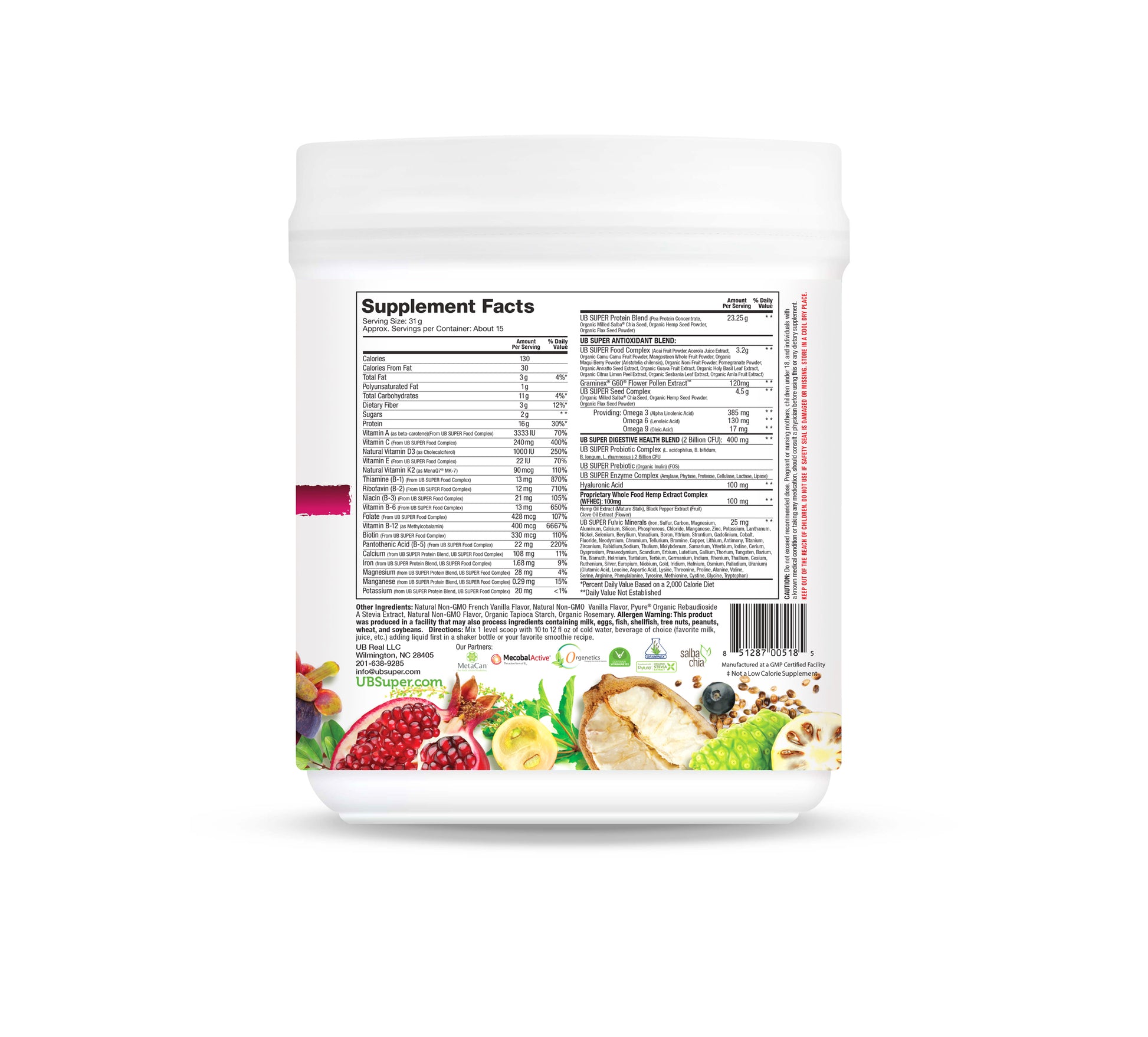This image depicts the back of a white plastic jar, which appears semi-transparent. The label, set in black text, is titled "Supplement Facts" at the top left corner. Below, two columns of small black writing detail the nutritional information, including serving size, servings per container, calories (notably 138), and other nutritional content. Towards the bottom of these columns, additional fine print and a barcode are visible, as well as the company's website, UBSoupSupper.com.

A range of colorful fruits and vegetables is vividly depicted at the bottom of the label, including what appear to be cherries, blueberries, a pear, a pomegranate, a coconut, and a lemon. There is also a small horizontal red line near the left center of the label. The image as a whole suggests that this could be a health-related product, possibly a protein powder or a blend of various nutritious ingredients, emphasizing a focus on wholesome and healthy eating.